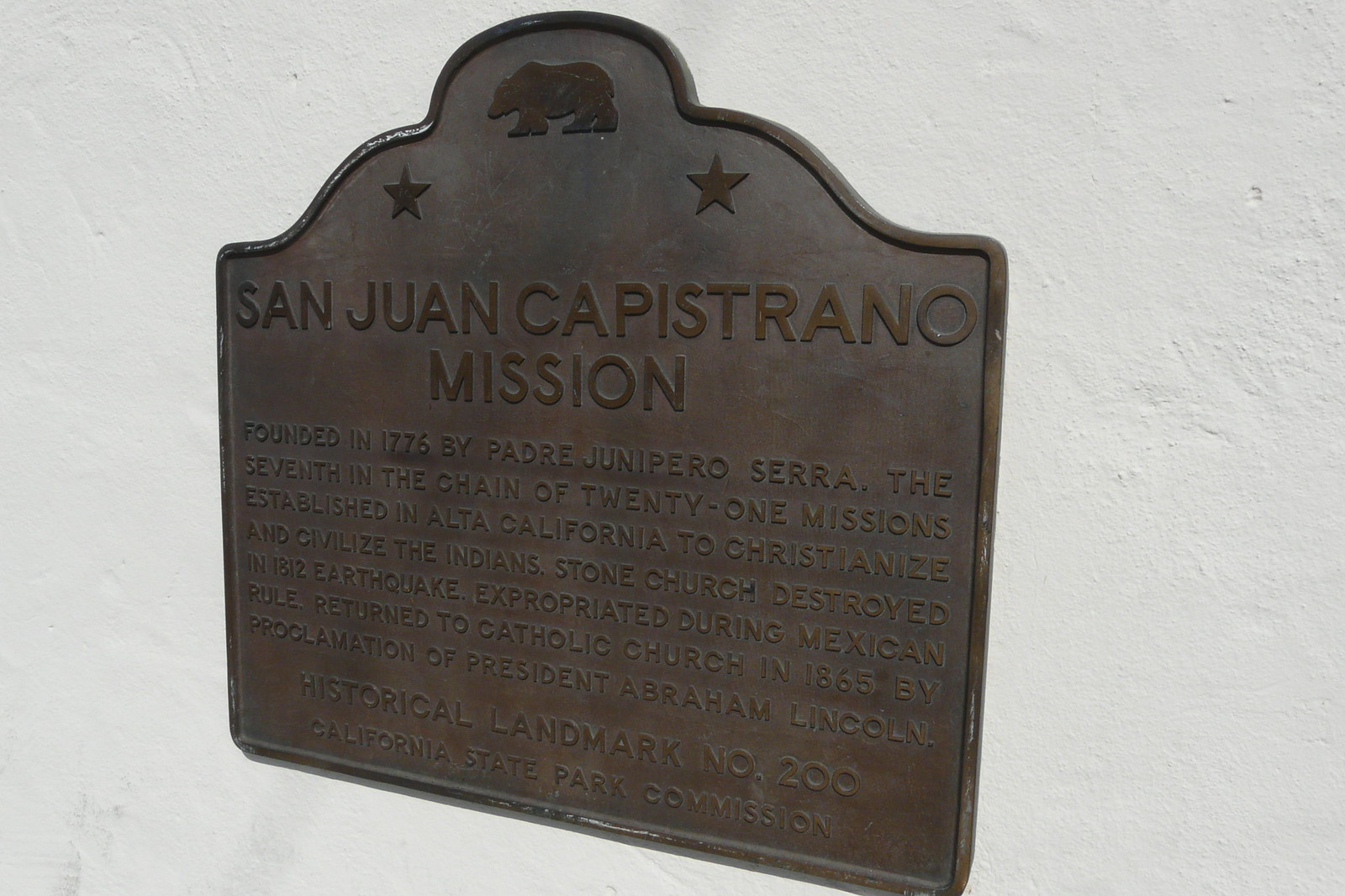The image depicts a historically aged, dark gray metallic plaque with a distinctive shape, being square at the bottom and sides, and rounded into a circle at the top. The plaque is mounted against a white wall. At the top center, there is an engraved symbol of the California bear flanked by two stars. Most prominent on the plaque are the large letters stating "San Juan Capistrano Mission." Below that, in smaller print, it details the historical significance: "Founded in 1776 by Padre Junipero Serra, the seventh in the chain of 21 missions established in Alta California to Christianize and civilize the Indians. Stone church destroyed in the 1812 earthquake, expropriated during Mexican rule, returned to Catholic Church in 1865 by proclamation of President Abraham Lincoln." At the bottom, the plaque indicates it is a "Historical Landmark Number 200," under the authority of the "California State Park Commission." The plaque exhibits some patina, particularly towards the bottom, indicating its age, though it remains in good condition overall.